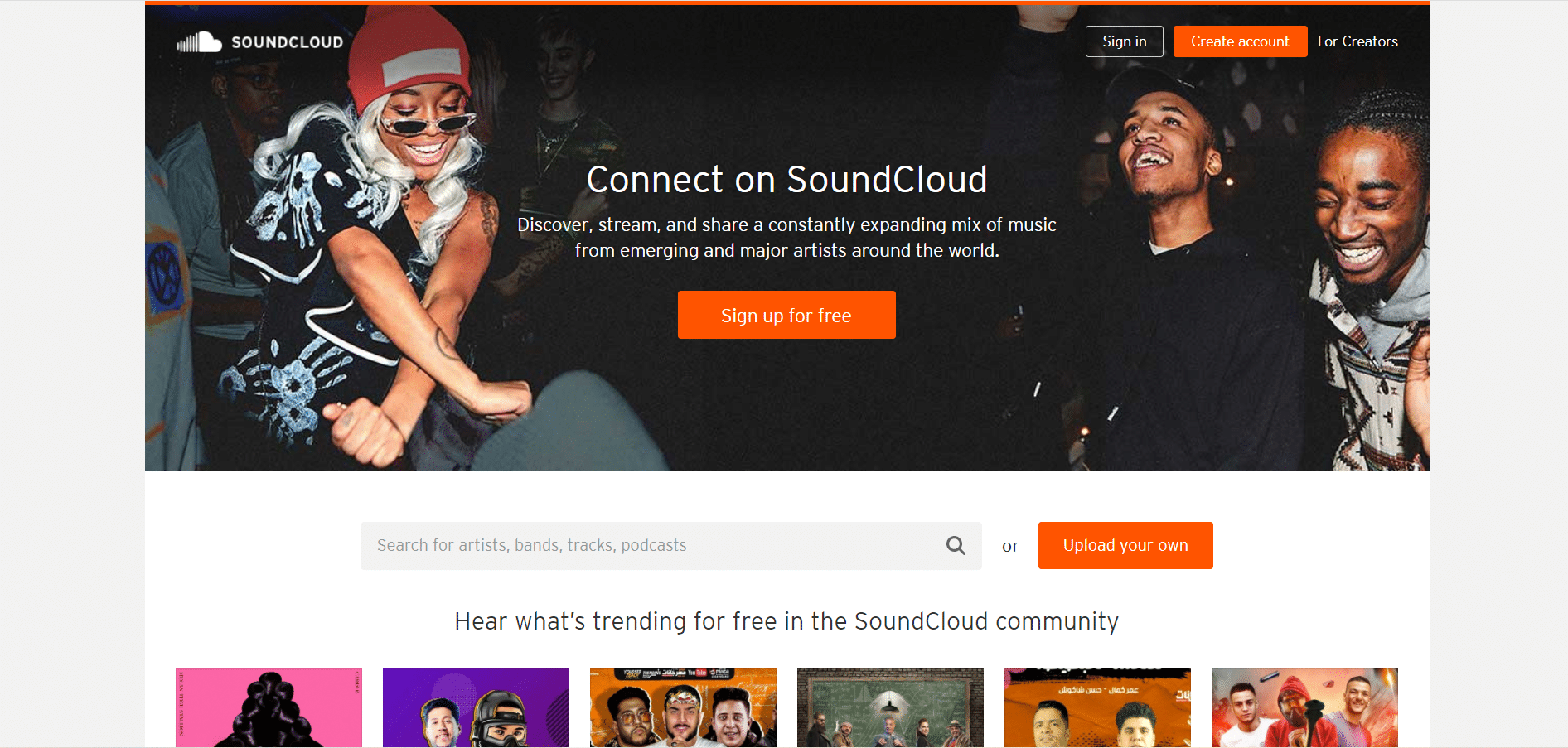In the image, the top part showcases a banner ad for SoundCloud, set against a predominantly black background. Below the banner is a vibrant snapshot capturing the essence of a lively party. The scene prominently features three African-American individuals, likely members of the hip-hop community judging by their attire.

On the left stands a young woman, likely in her early twenties, wearing a striking red knit hat adorned with a white rectangle. She sports chic shades and a white-blonde wig, which contrasts with her black shirt and dark pants. A visible tattoo graces her arm, adding to her edgy look.

To her right are two young men. The first, wearing a black baseball cap and a matching long-sleeve shirt, stands beside another individual with braids, dressed in a multicolored shirt. All three are smiling brightly, radiating a sense of camaraderie and joy.

Centrally placed within the picture, the text "Connected on SoundCloud" invites viewers to sign up for free, highlighted by an orange button. Below this call to action is a search bar for exploring artists, bands, tracks, and podcasts, marked by a magnifying glass icon for easy access.

At the bottom of the image, "Here's what's trending for free in the SoundCloud community" introduces a collection of six album covers, presumably from independent artists, emphasizing the platform's support for emerging talent.